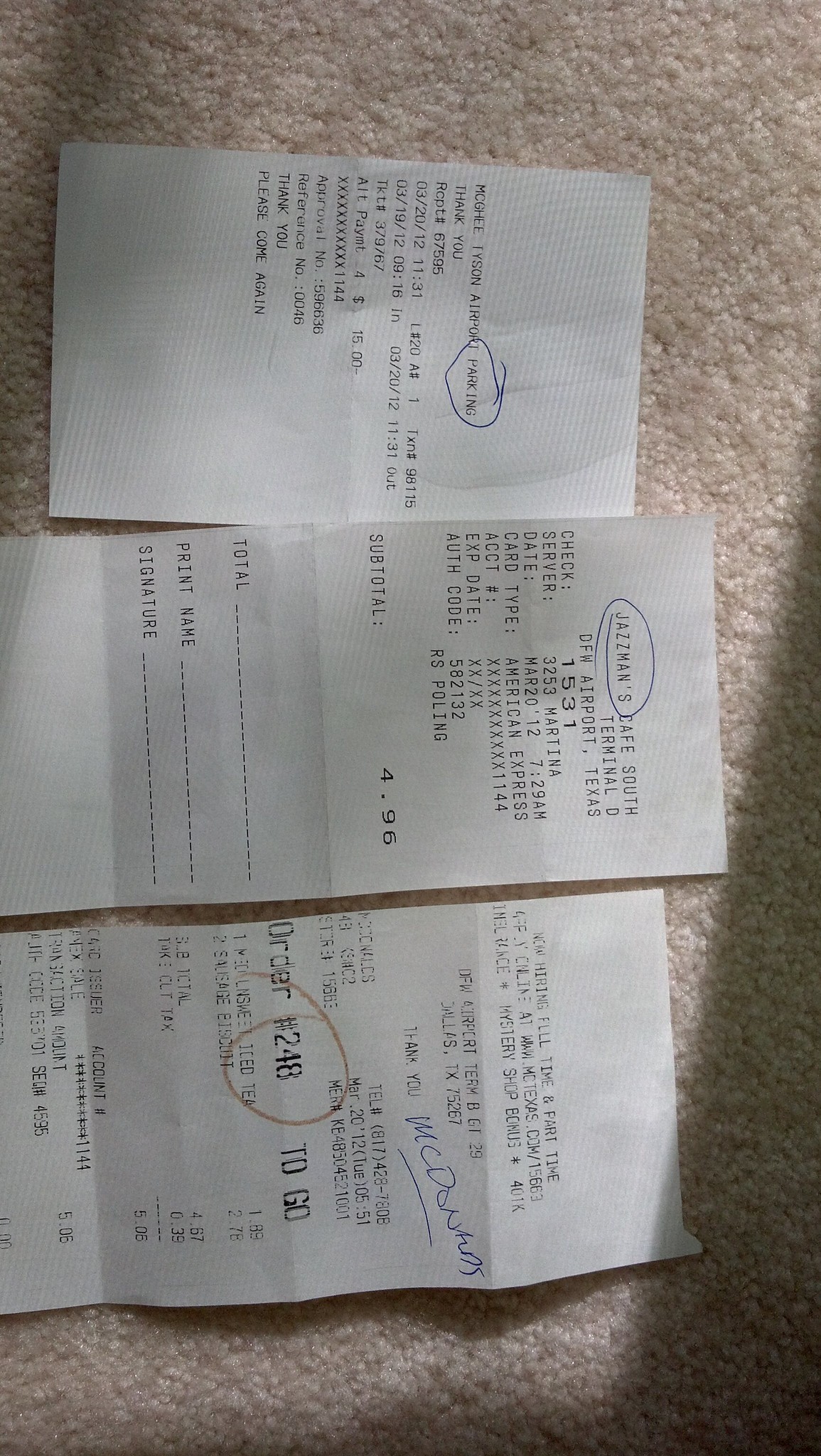A detailed caption of the image depicts three receipts lying horizontally on a beige carpeted background, rotated 90 degrees clockwise. The image encompassed subtle shadows primarily in the upper right-hand corner. From a standard viewing orientation, the far left receipt originates from McGee Tyson Airport Parking, highlighting an amount paid—$15—with the word "Parking" circled. The middle receipt belongs to Jasmine's Cafe located in Terminal D, with "Jasmine's" also circled and reflecting a total of $4.96. To the far right, the third receipt, though difficult to fully decipher due to print quality, advertises job openings for full and part-time positions at an airport. It contains references to DFW (Dallas/Fort Worth International Airport) and the city of Dallas, Texas. Handwritten in blue pen on this last receipt is "McDonald's," with "Order Number 24B" circled in brown pen or pencil.